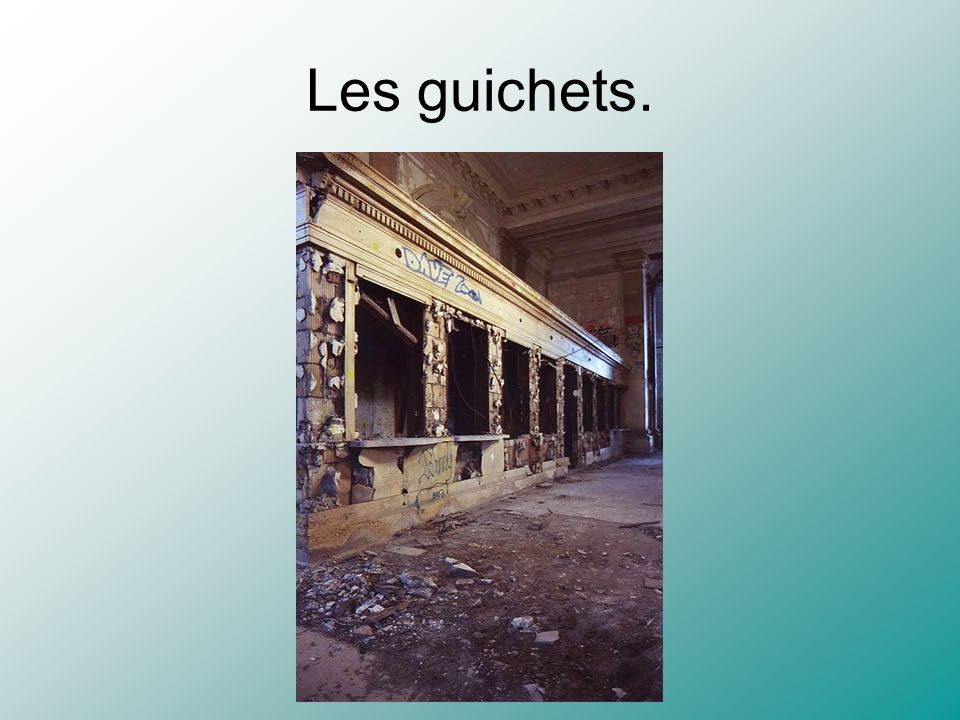The image captures an abandoned, dilapidated building interior with high, intricately designed stone ceilings, now deteriorating. Broken stones and torn-up flooring litter the ground, depicting a once beautiful structure now in ruins. Mounted on a gradient background fading from white to dark teal at the bottom right, the image features graffiti, including the name "Dave" in blue, scrawled on a small alcove or kiosk structure extending from the wall. The words "LES GUICHETS" in black sans-serif font are prominently written at the top center of the slide-like presentation. Natural light streams in, complementing the artificial light that falls from the ceiling above, illuminating the scene.